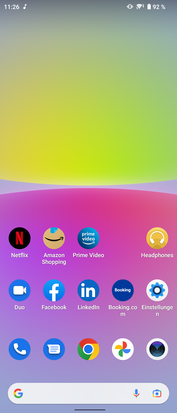This vertical rectangular image appears to be a screenshot from a cell phone. At the top left corner, it displays the time "11:26" in a white font. On the right side, it shows the battery life as "92%," with a filled battery icon to its left.

The image background begins with a gray section at the top, transitioning into various colors: a yellow-gold hue on the left, blending into a green hue on the right, both slightly blurry. The middle portion of the background is a small lavender area, and the bottom section transitions from hot pink to lavender, particularly on the lower left-hand area.

The bottom section, embellished with logos or icons for various applications, includes both the icon and the app name under it. From left to right:

- Netflix: a black circle with a red "N".
- Amazon Shopping: a tan circle with a black arrow pointing to the right and a touch of blue at the top.
- Prime Video: a turquoise circle with "Prime Video" written inside in white.
- A yellow circle with a pair of white headphones, labeled "headphones."

Below these, from left to right on the second row:

- Duo: a bright blue circle with a camera icon and "Duo" written underneath.
- Facebook: a bright blue circle with a lowercase "f" and "Facebook".
- LinkedIn: a medium blue circle with a lowercase "in" and "LinkedIn".
- booking.com: a dark blue circle with "booking.com" written in white.
- An unreadable turquoise circle with a central white dot surrounded by black, creating a star-like pattern.

The last set of icons, which do not have any accompanying text, include:

- A blue dot with a white phone icon.
- A blue dot with a piece of white paper.
- A swirl of red, green, yellow, and a blue dot.
- A white circle featuring a pinwheel flag in red, yellow, green, and blue, resembling a four-leaf clover.
- A white circle with three-quarters black and a purple top.
- A horizontal oval white bar with a "G" on the left-hand side.